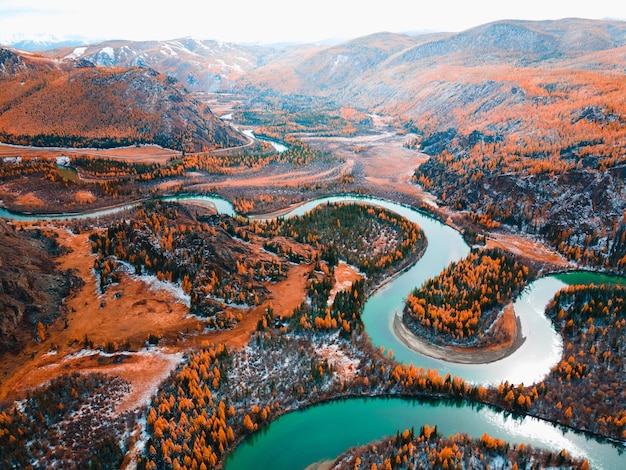This striking image, which could easily be mistaken for an extraordinary painting or a professional aerial photograph, captures a breathtaking autumnal landscape. The focal point is a meandering river, reminiscent of a sinuous snake, weaving through a vivid tapestry of natural elements. The water, in shades of greenish-blue, contrasts beautifully with the surrounding rusty copper and green mountains and hills. These mountains are dotted with a dense forest of trees showcasing autumn foliage in a plethora of hues—predominantly orange, with splashes of red and yellow, and various shades of brown, indicating the fall season. The sky above is predominantly white, interspersed with hints of blue and wispy clouds, adding depth to the scene. The expansive view reveals a complex interplay of crisscrossing water bodies and vividly colored tree lines, creating an almost surreal and otherworldly presentation of nature's beauty, all devoid of human presence or text.